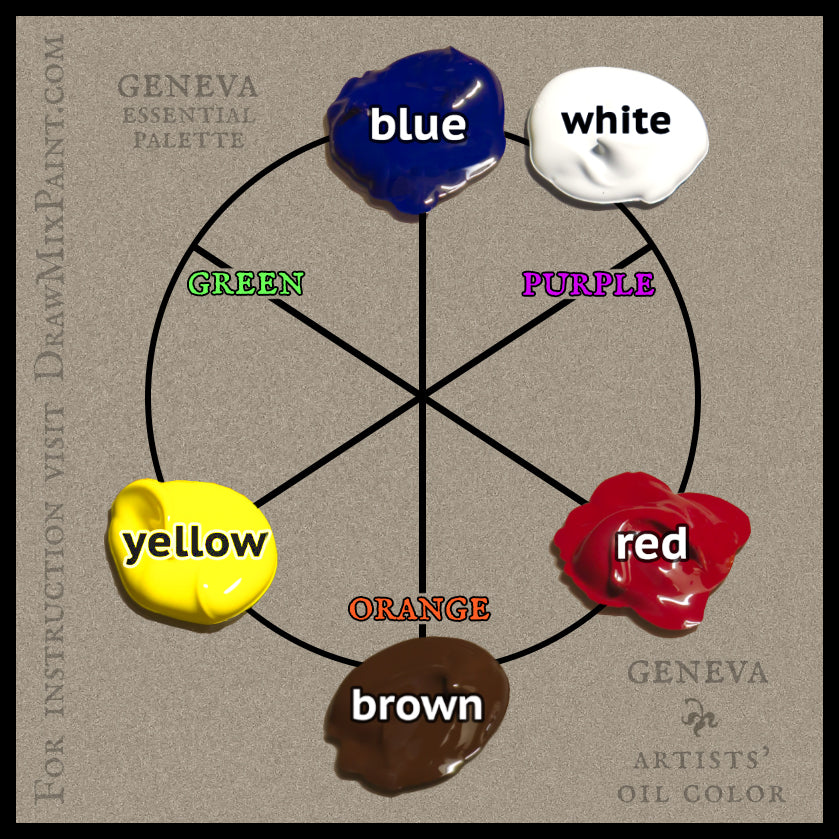The image displays a Geneva Essential Palette, designed to instruct on color mixing. The background resembles dark brown or gray stone-textured paper or a digitally created cardboard craft surface. Dominating the image is a circle divided into six segments like a pie chart, bordered by plain black line art. Each segment contains splotches of different paint colors—blue, white, red, brown, and yellow—with corresponding labels. 

The circle features additional labels for secondary colors: green (between blue and yellow), purple (between blue and red), and orange (above the brown splotch). Text instructions are included, with "For instruction, visit drawmixpaint.com" running vertically along the side. "Geneva Essential Palette" and a Geneva leaf symbol mark the bottom right corner, identifying the artist's oil color brand. The arrangement demonstrates basic color mixing principles, such as blue and yellow creating green, aligning with the labeled secondary colors.